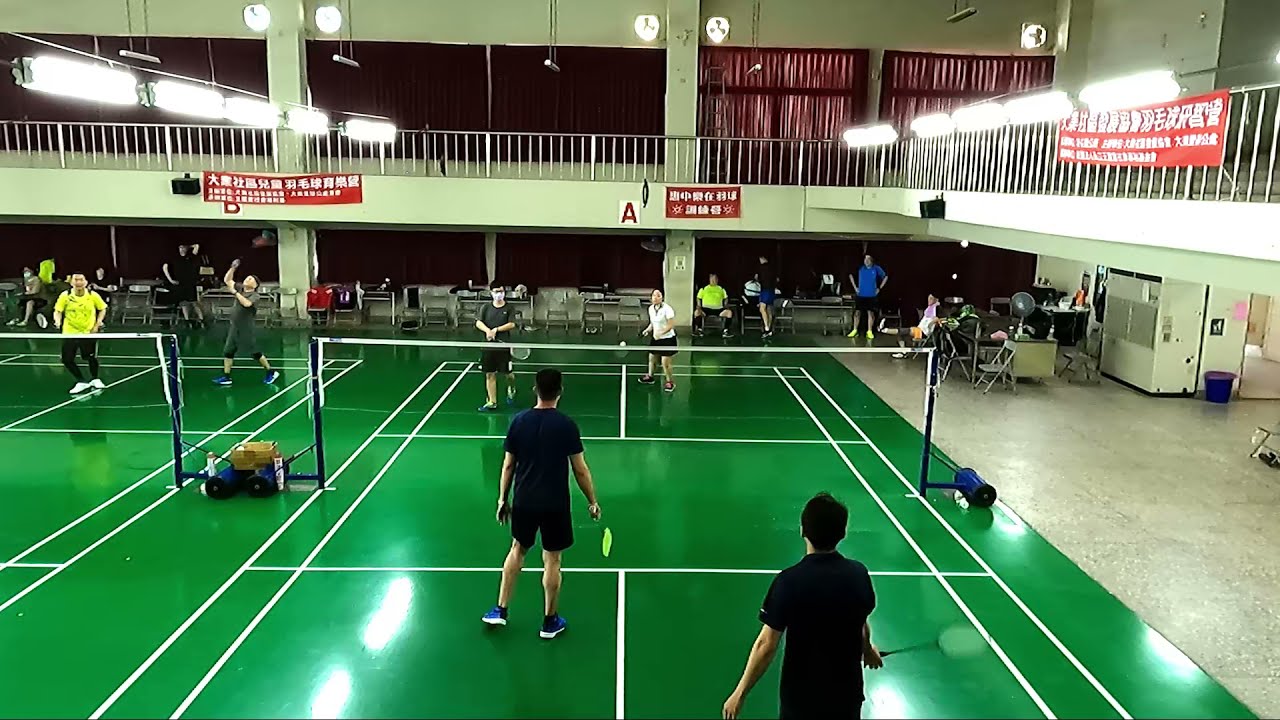This photograph captures a vibrant scene inside a large, brightly lit sports center, specifically focusing on indoor badminton courts. The image is taken from an elevated position, providing a comprehensive view of the setup. The sports center features white walls adorned with red curtains over large windows, giving a glimpse of the dark exterior outside. Red banners, featuring what appears to be an Asian language, hang from the metal railings of a mezzanine level that stretches from left to right and diagonally from front to back on the right side.

The flooring is a vivid green marked with white striping for the badminton courts. Blue nets with wheeled poles are positioned across each court. At the center of the frame, two men in black shirts and shorts are engaged in a match, facing a duo across the net consisting of one person in a white shirt and another in gray. To the left, another court is partially visible, showing two men opposite each other, one in a yellow shirt and the other in gray.

Spectators are scattered along the walls, some sitting and some standing, attentively watching the players. There is a desk to the right with what seems to be an air conditioning unit or some other type of conduction equipment nearby. Doors and hallways are also visible on the far right. The detailed setup and bustling atmosphere suggest an organized event, bringing together players and onlookers in an immersive and active environment.